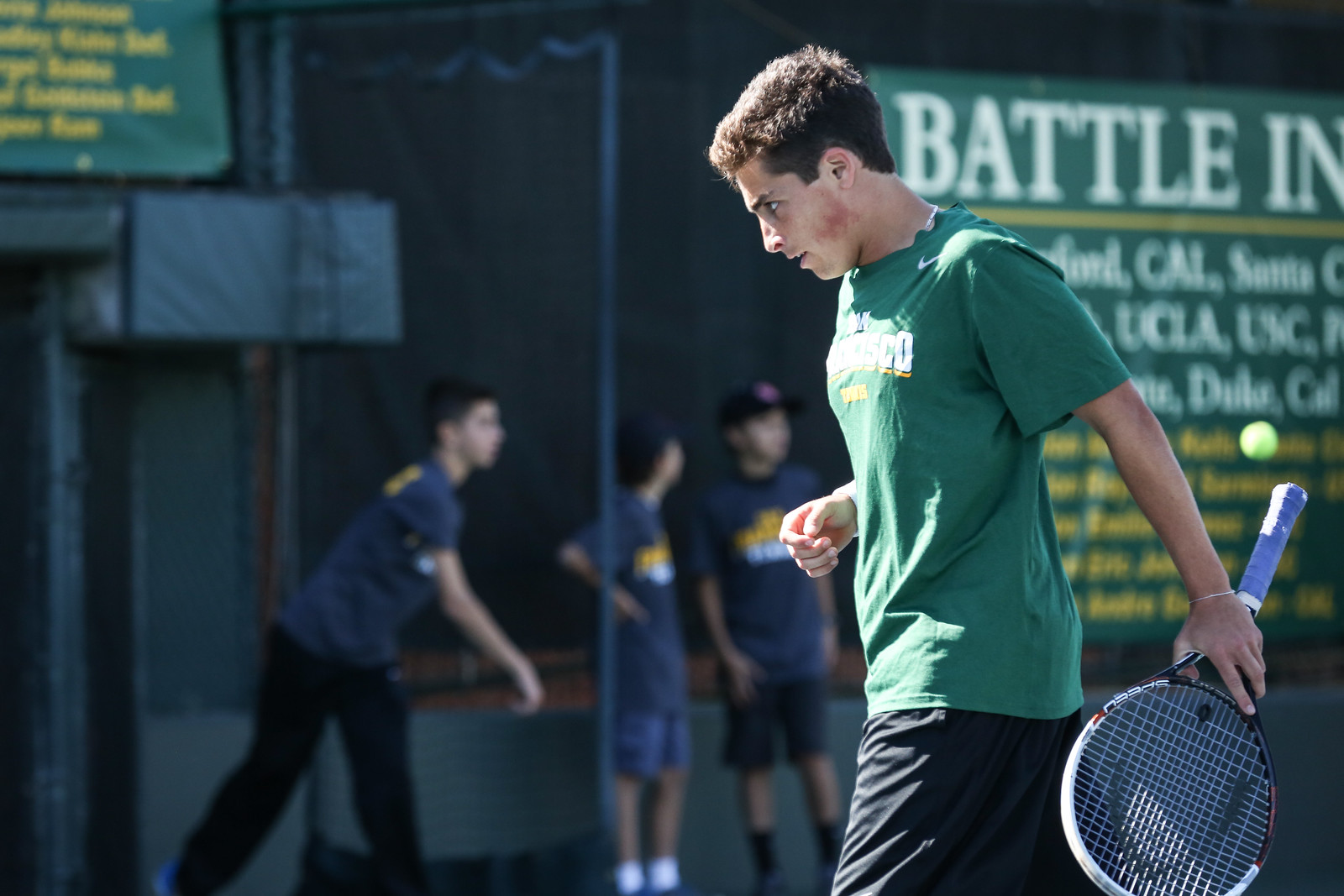In the photo, a young man with short, dense brown hair is captured in a side profile as he walks forward, one leg in front of the other. He is wearing a green t-shirt and dark shorts, and is holding a tennis racket by the neck in his left hand. The sunlight illuminates his chest, highlighting that he is outdoors, possibly on a tennis court or sports arena. In the background, three younger boys in matching dark gray t-shirts and shorts stand together, seemingly engaged in a sport. A green and white sign, partially obscured with the text "Battle Inn," is also visible. The background is somewhat dark and blurry, adding contrast to the well-lit foreground. There are draping and poles situated between the young man and the sign, and a tennis ball can be seen behind him, further indicating the sports setting.